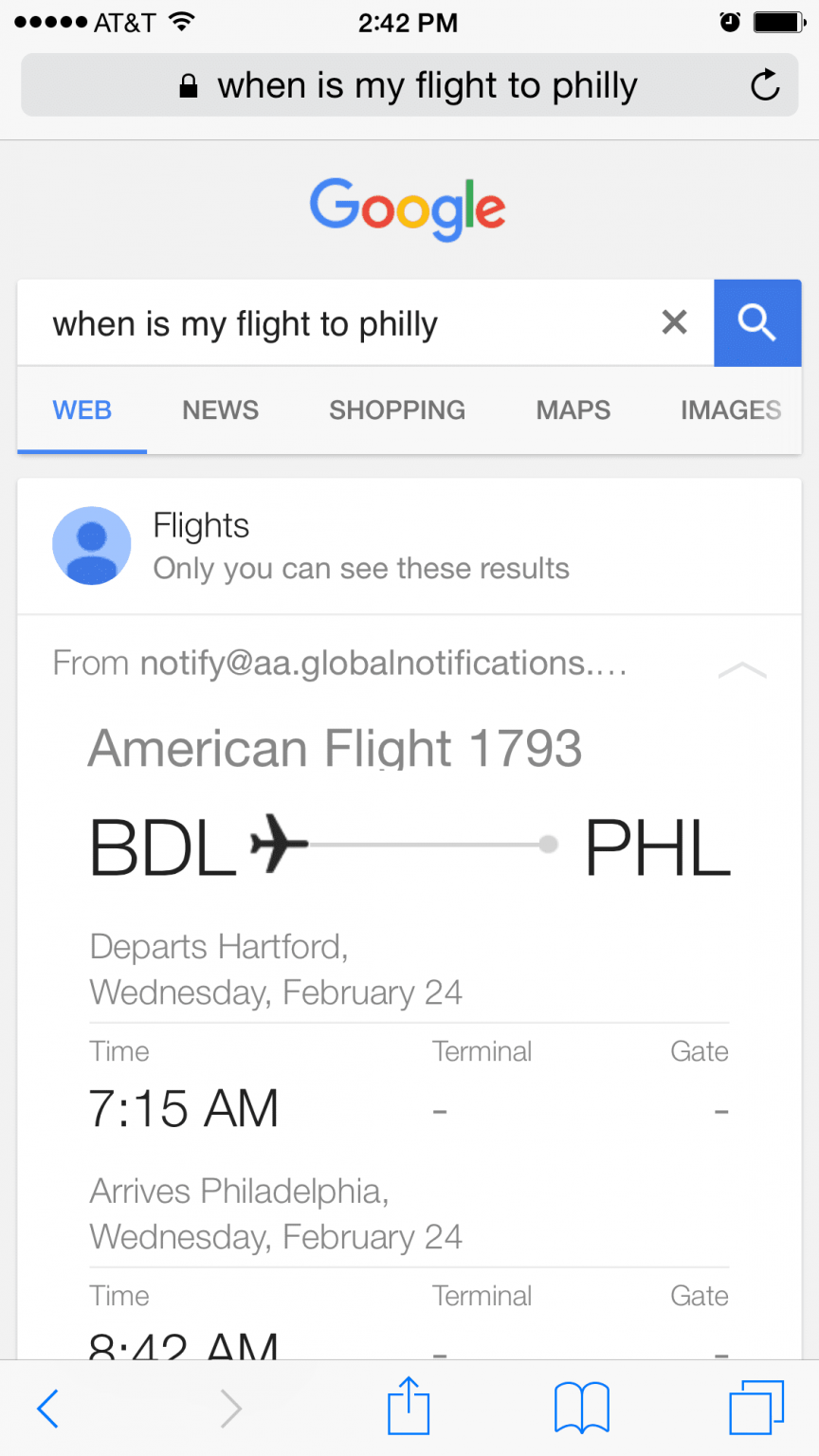Screenshot from a smartphone displaying an internet search result regarding a flight:

**Upper Section of the Screen:**
- **Status Bar (Top Left to Right):** Five black horizontal dots indicating signal strength, "AT&T" carrier name, Wi-Fi icon, current time "2:42 PM," alarm icon, battery icon mostly full.
  
**Search Bar:**
- **Text:** "when is my flight to Philly" with a lock icon on the left and a circular arrow on the right.
- **Google Branding:** The word "Google" with its letters in different colors (capital "G" in blue, first "O" in red, second "O" in yellow, lowercase "g" in blue, "l" in green, "e" in red).

**Search Result Section:**
- **Query Repeated:** "when is my flight to Philly," with a gray 'X' icon to clear the search and a blue button with a magnifying glass to initiate the search.
- **Headers:** Options for "web," "news," "shopping," "maps," "images."
- **Flight Information:** 
  - Personalization Note: "Only you can see these results."
  - Notification Source: "notify at AA.global notifications"
  - Flight Details: "American Flight 1793"
    - **Route:** "BLD" (departure) → "FHL" (destination) with an airplane icon.
    - **Departure Info:** "Departs Hartford, Wednesday, February 24th, 7:15 AM, Terminal Gate"
    - **Arrival Info:** "Arrives Philadelphia, Wednesday, February 24th, 8:42 AM, Terminal Gate"

**Bottom Section of the Screen:**
- **Navigational Icons:**
  - Blue arrow pointing left (back button)
  - Gray arrow pointing right (forward button)
  - Box with an arrow pointing up (share button)
  - Open book icon (reading mode)
  - Two overlapping squares (tabs feature).